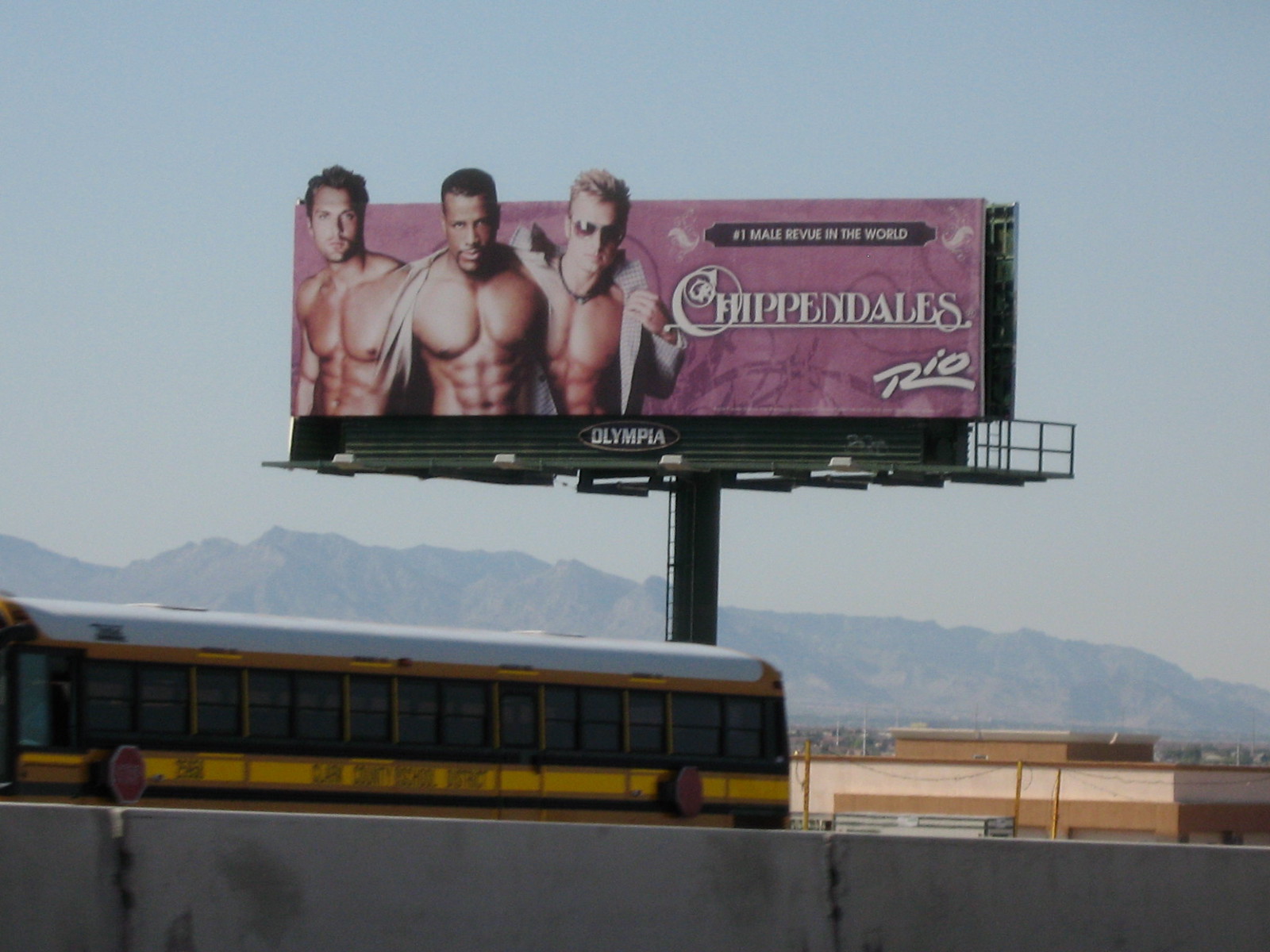In this roadside scene, a large, yellow and black school bus with a white top navigates past a concrete wall that divides the lanes. In the background, a substantial factory building constructed of brown brick and topped with white accents stands prominently. Beyond the industrial structure, a mountain looms under a grayish sky, adding depth to the landscape. A striking billboard catches the eye on the side of the road; cut out in the shape of three heads, the sign advertises "Chippendales in Rio." The billboard, hued in purple, features images of three shirtless, muscular young men, enhancing the vibrant yet rugged atmosphere of the scene.